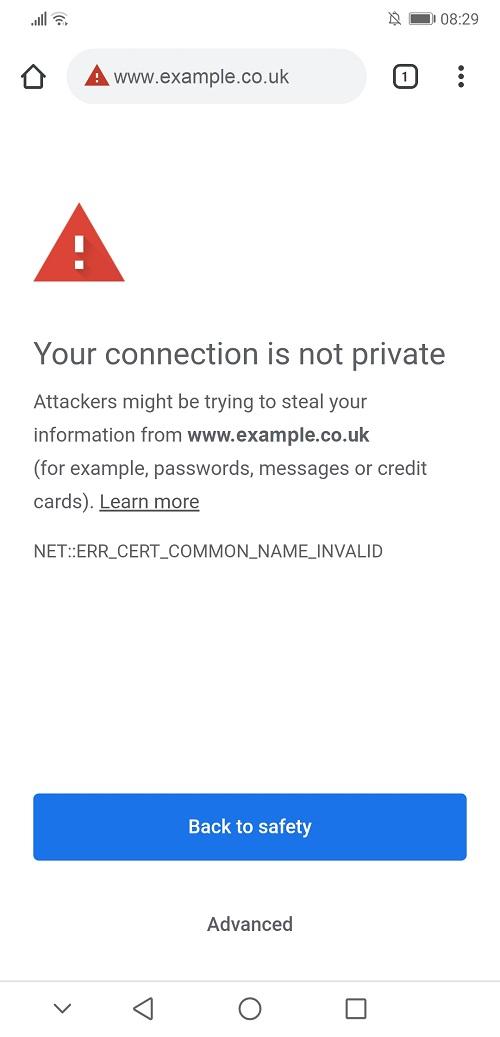The image depicts a smartphone screen displaying a security warning from a web browser. The status bar at the top of the screen shows a full signal indicator, silent mode (sound turned off), and an almost fully charged battery at 8:29. The main content of the screen reveals a warning message with a small house icon next to the URL "www.example.co.uk". To the left of the URL, there is a red triangle with a white exclamation point, indicating a security issue.

Next to the triangle, there's a black square with the number "1" inside. Below the URL, three horizontal black dots signify additional options or settings. The primary warning message is prominently displayed with another red triangle and white exclamation point. The text in black states: "Your connection is not private. Attackers might be trying to steal your information from www.example.co.uk, for example, passwords, messages, or credit cards."

Below the warning text, there is a clickable, underlined link that reads "Learn more." The error code "NET::ERR_CERT_COMMON_NAME_INVALID" is provided beneath the link, highlighting the specific security issue. At the bottom of the screen, there is a large blue button labeled "Back to safety," and below it, a smaller option labeled "Advanced."